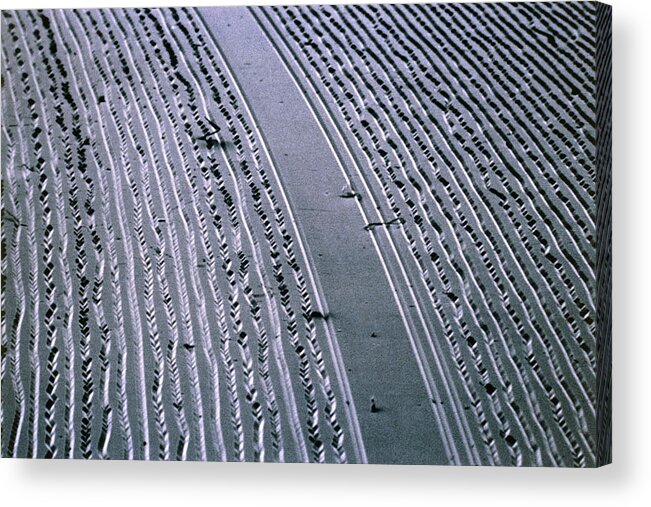The image is a black and white abstract photographic print displayed on a canvas, featuring an intricate assortment of grooves and lines that resemble a blend of carved and chiseled patterns. The composition is dominated by parallel lines interspersed with zigzag and fabric-like textures. These lines originate from the bottom and curve upward, with variations in their direction and spacing across the image. Smaller grooves are present on the left and right sides, while a prominent groove runs through the center, evoking the appearance of a street. The broader central section and adjacent thinner lanes exhibit a distinct gray hue. The right edge of the image is marked by a border featuring what looks like thread-like lines descending from the top to the bottom. The overall texture conveys a sensation akin to a chisel carving through wood, dense with a variety of line qualities and intensities. The print’s noisy texture and the grooved patterns contribute to its complex, abstract nature, giving the impression of being meticulously crafted and sold as contemporary art.